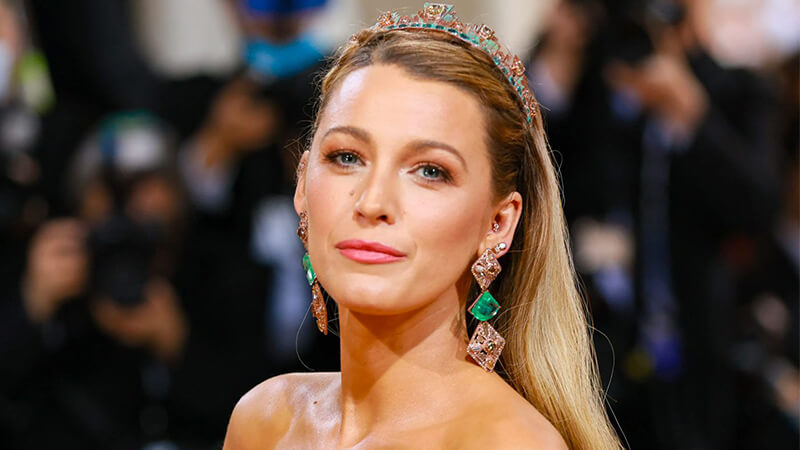This photograph features Blake Lively, a well-known American actress, dressed elegantly for an event. The image is cropped at chest level, highlighting her face and upper torso. Blake has long, flowing blonde hair, partially held back by a headpiece that resembles a tiara or crown, intricately decorated with shades of green, olive, and gold. Her makeup is understated yet striking, with light pink lipstick and well-defined brown eyebrows complementing her blue eyes. 

Her ears are adorned with elaborate, dangling earrings composed of three diamond-shaped sections: a gold one at the top, followed by a green one, and another gold one at the bottom. Blake's strapless outfit suggests a glamorous, off-shoulder dress, though the actual garment is not fully visible due to the cropping of the photograph. She is centered in the image, looking directly into the camera with an air of confidence and poise.

In the blurred background, photographers and possibly audience members can be seen, suggesting that this photo was captured at a high-profile event or red carpet appearance, with the crowd's dark clothing providing contrast to her luminous presence.